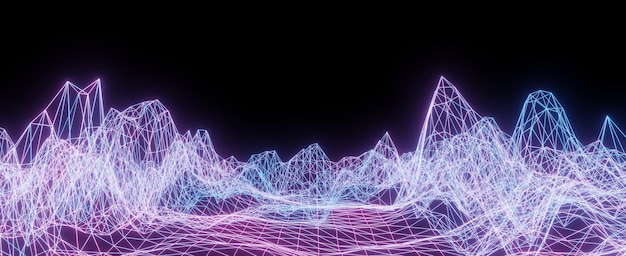A striking image features a predominantly black background, giving it a sleek, nearly void-like appearance. Set against this dark backdrop is an intricate, computer-generated design that evokes a blend of cyberpunk and 1980s computer graphics. Interwoven patterns in white, purple, light blue, and hints of pink form geometric, topographic-like peaks and waves across the lower half of the image. These lines create a glowing mesh grid reminiscent of a spider's web, with various points converging into sharp peaks and rounded mounds. The highest peak, predominantly purple, stands on the right side of the image, detailed with an array of intersecting lines that form triangles, diamonds, squares, and rectangles. This dynamic composition of colors and shapes gives the impression of a flowing, mountainous landscape suspended in a digital void.